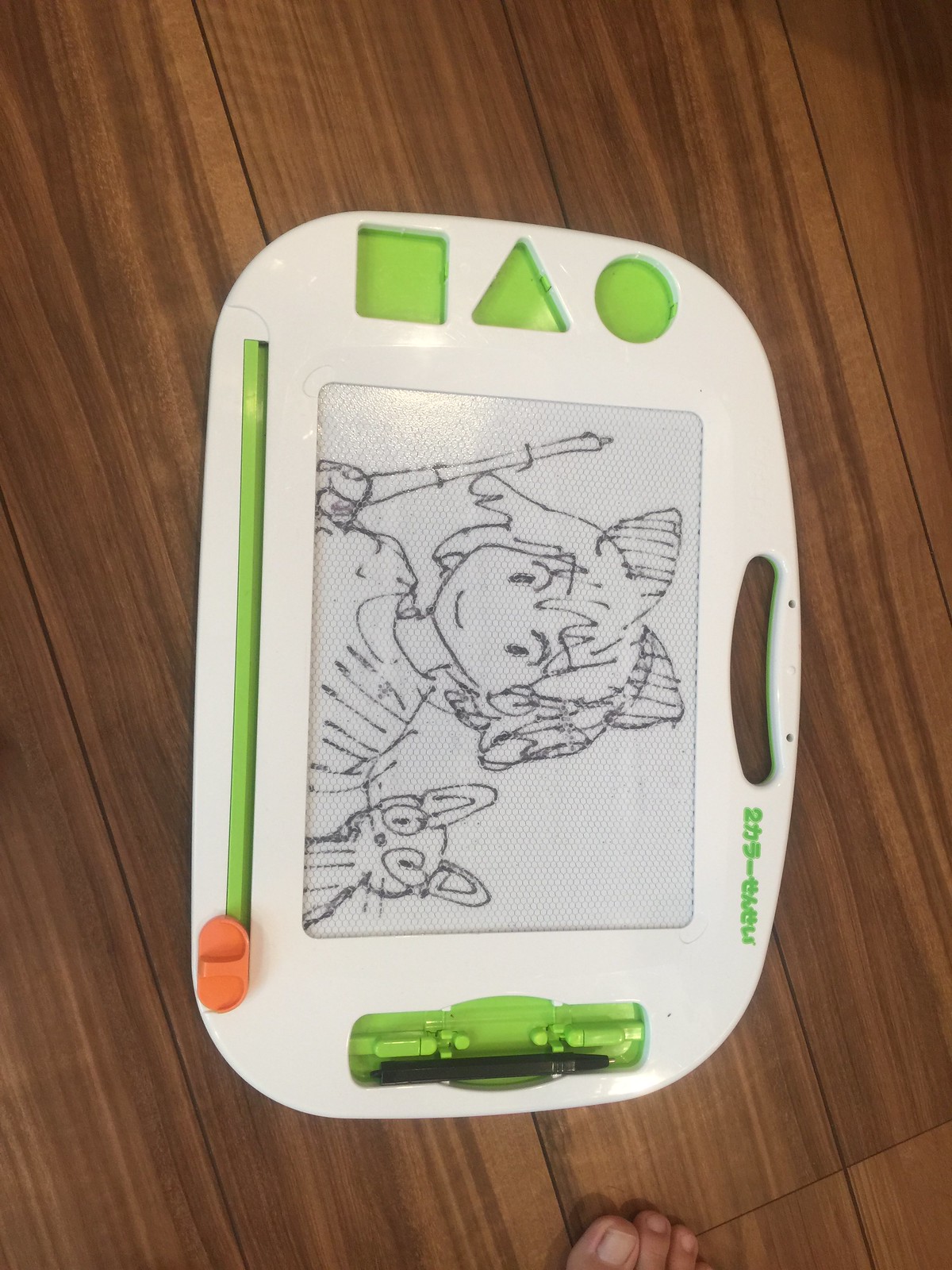In the photograph, a children's magnetic drawing board is placed on a wooden textured floor, slightly tilted so that viewers need to turn their heads to see it properly. The board features a white top layer with lime green accents, including green shapes like a circle, triangle, and square, which have missing pieces. The drawing board has a handle at the top and an orange slider used to erase the drawings. There is also a holder for the magnetic pen. Japanese lettering can be seen near the handle. The board has a whimsical drawing of a girl with a bow in her hair holding a stick, accompanied by a cat with large ears on her right. At the bottom of the image, part of a person’s toes is visible, providing a sense of scale to the setup.